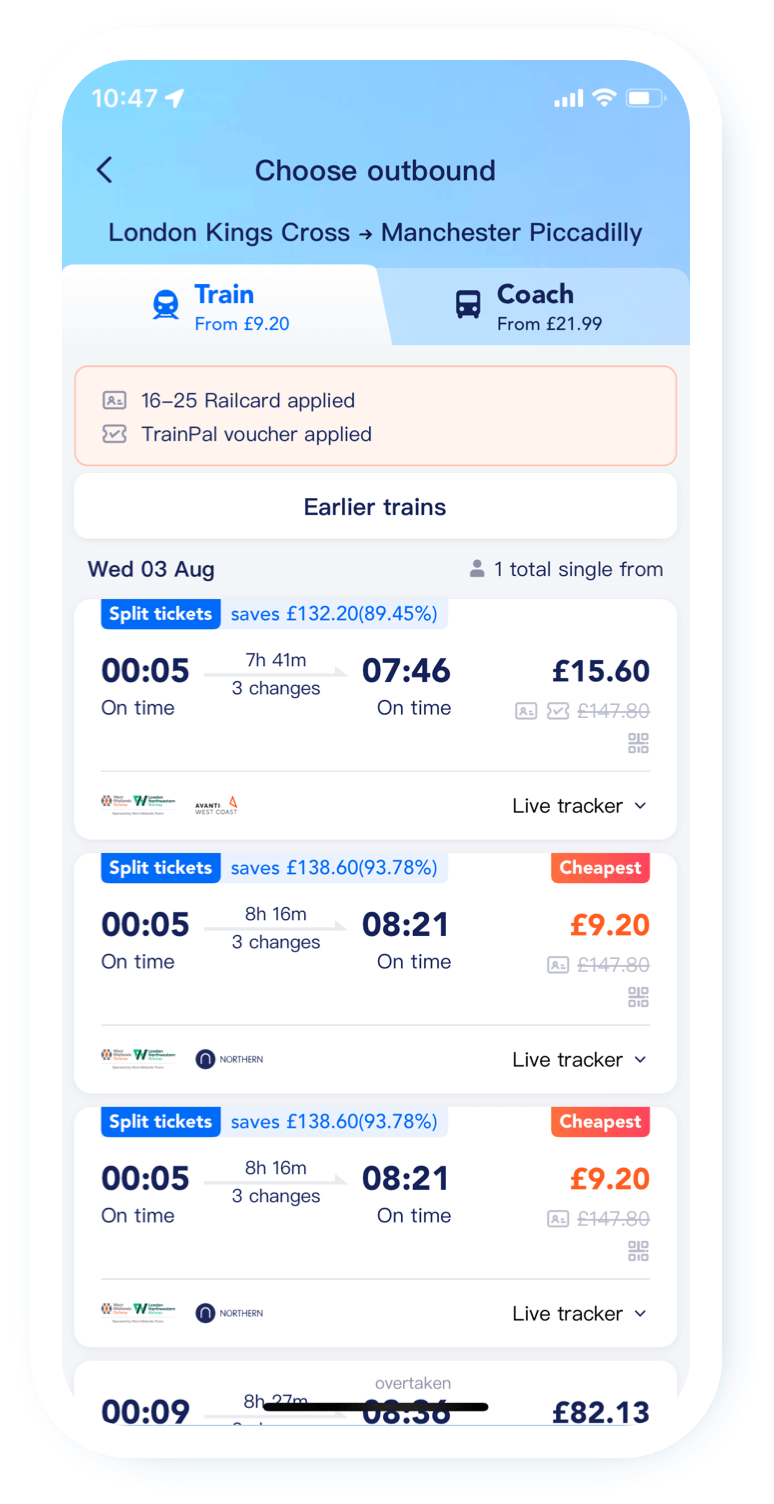The image is a screenshot from a mobile transportation application, specifically depicting travel options within the United Kingdom. The top part of the image displays toggles for selecting either train or coach travel, with prices starting from £9.20 for trains and £21.99 for coaches. The journey in question is from London Kings Cross to Manchester Piccadilly. At the very top, it shows an option to "Choose Outbound" journey details.

Additionally, a 16 to 25 Railcard discount is applied, alongside a "train power voucher," indicating that various discounts are being utilized. Below these options, multiple travel times and dates are listed for train journeys. Notably, the original fare for these trips is £147.80, but thanks to the applied discounts, the prices have been significantly reduced to as low as £9.20 and £15.60. Each heavily discounted price is prominently displayed with a strikethrough on the original fare, highlighting the substantial savings available through the app.